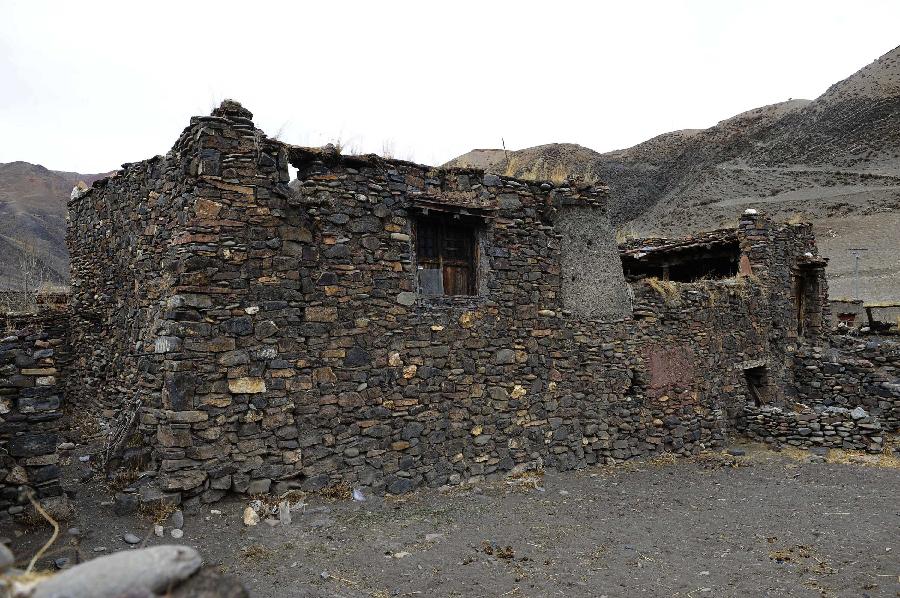The photograph captures a dilapidated stone building situated in a rugged, mountainous desert environment. The structure is primarily composed of varied stone pieces, ranging in colors from light gray to dark charcoal, blending seamlessly with the surrounding arid landscape. The terrain slopes upward from the base of the building, leading towards the mountainous ridges that dominate the background. A small window punctuates the long side of the building facing the camera, while the short side and a corner of the structure are visible to the left. A significant section of the wall on the right appears to have been cut away, with part of the roof missing, suggesting significant damage or decay. The bright daytime sky above is almost pure white, providing a stark contrast to the earthy tones and enhancing the clear, detailed view of the scene. Scattered patches of brown plants and sparse grass add to the desolate atmosphere, emphasizing the isolation and age of the stone edifice.